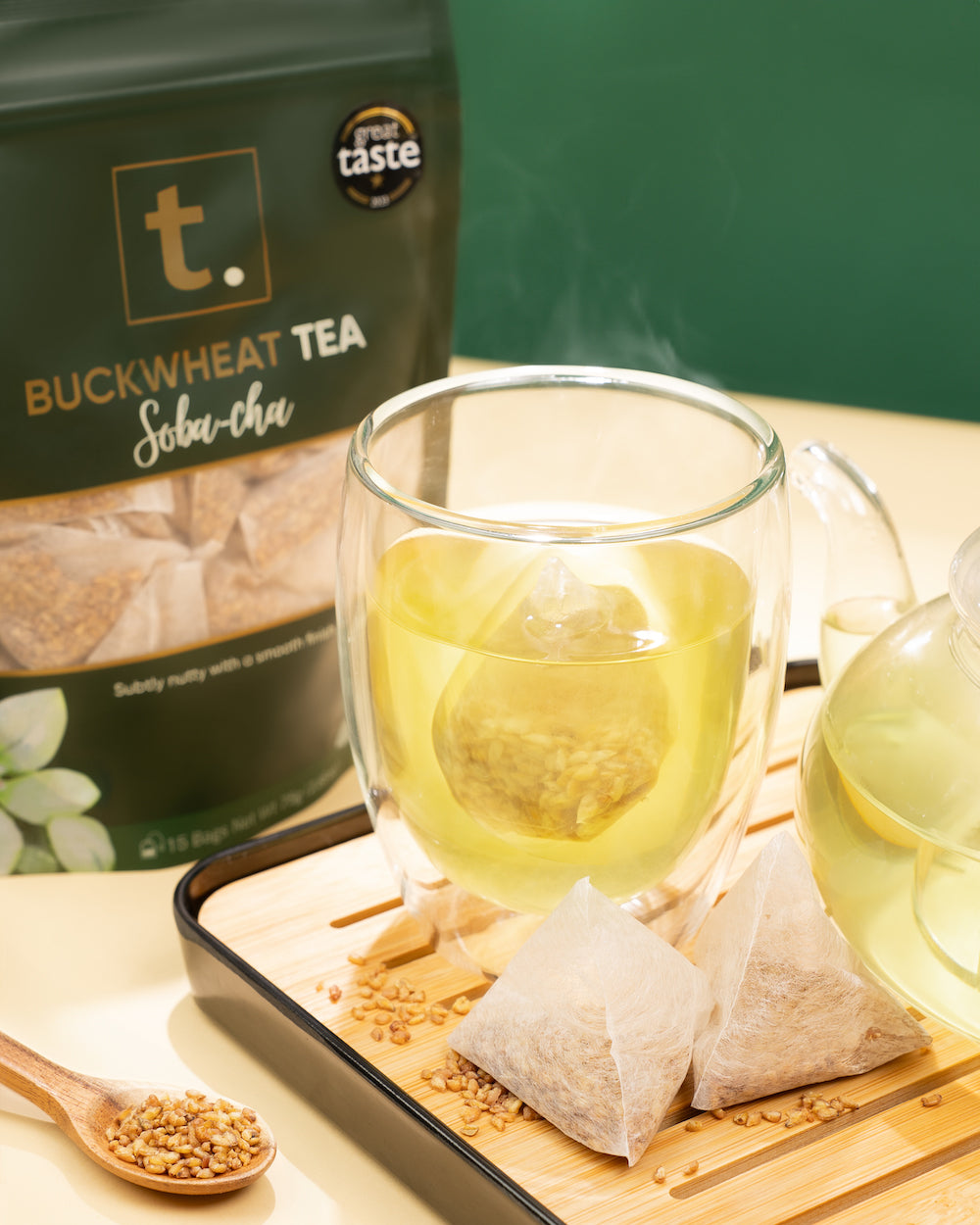A product advertisement and food blogger's photograph of a bag of buckwheat tea, specifically "Soba Cha," featuring prominent elements on a green-themed background. Central to the image is a green tea packet with a black logo reading "Great Taste," and a yellow square box displaying "tea" in golden letters, below which it says "buckwheat tea, Soba Cha." The tray in the foreground is black with a wooden base, holding a glass cup filled with light yellow tea, similar in color to mel-y-ellow lemonade, alongside a matching glass teapot. Scattered around are brown and tan buckwheat seeds, some placed in a wooden spoon at the bottom left corner. Additional large tea bags with seeds are also present on the tray. In the background, a brown plastic bag reiterates "tea. buckwheat tea, soba cha," enhancing the product's branding.